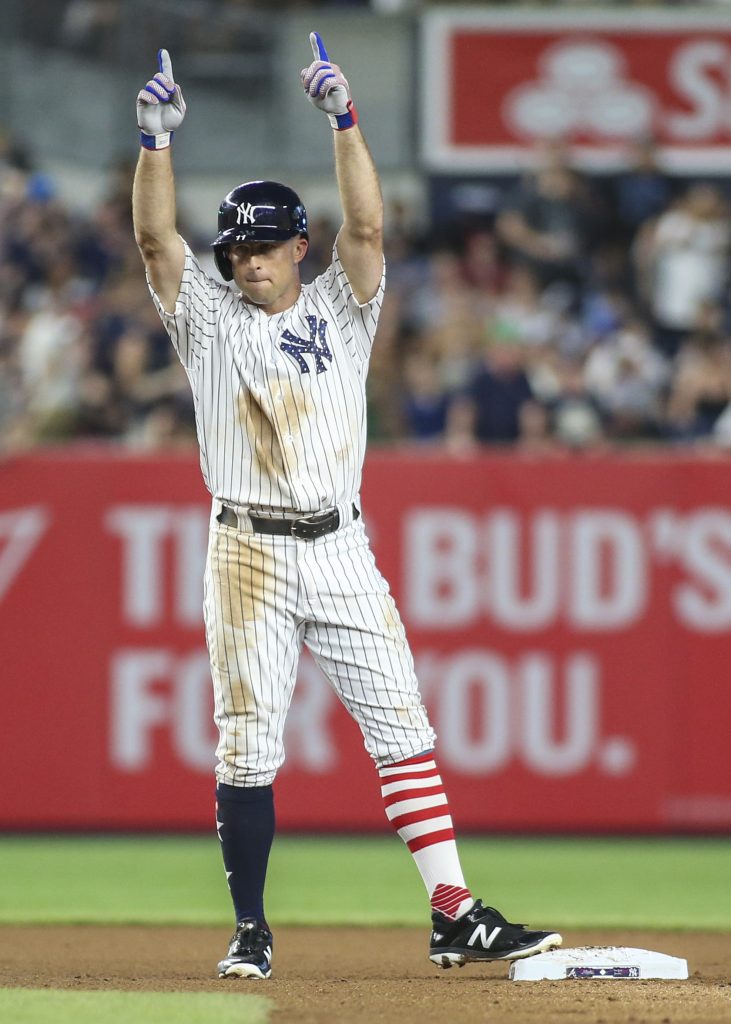A jubilant New York Yankees player, clad in the iconic white pinstriped uniform with the interlocking navy blue "NY" logo, stands triumphantly with one foot on a base. His black sneakers, marked with an "N" on the side, are firmly planted as he raises both arms above his head in celebration, likely signaling a successful hit. The uniform bears evidence of a competitive game, with brown dirt stains from a slide. He sports gray gloves accented with red and blue, and a navy-blue Yankees cap featuring the team's logo. Behind him, a "This Bud's for you" advertisement is prominently displayed, blending into a vibrant scene filled with a sea of excited fans, indicative of a sold-out night. The lush green grass and the well-trodden baseball dirt frame this moment of triumph, highlighting the player's jubilant stance at the base.